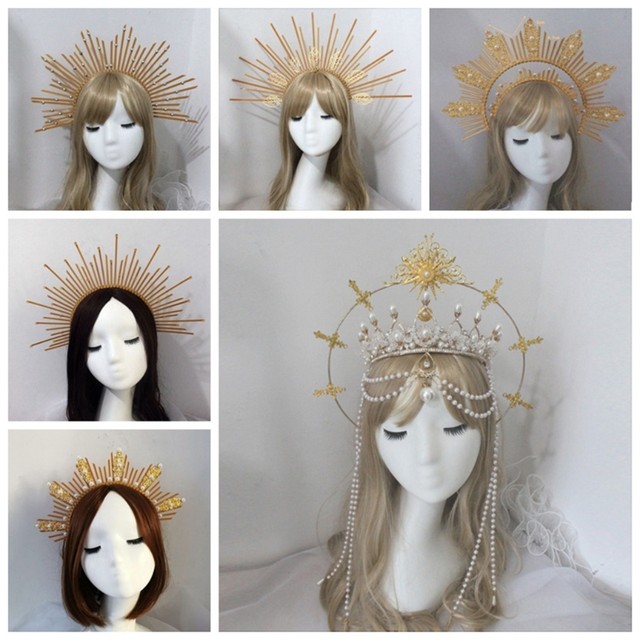This image showcases six detailed mannequin heads used for wig displays, each adorned with intricate headpieces. Arranged in a grid-like fashion, the top row features three one-inch by one-inch images of white-skinned mannequins with distinct hairstyles and headpieces. The mannequin on the far left has a sunburst-themed crown with alternating lengths of bursts, light brown hair, and prominent black eyebrows. The middle mannequin sports long silver-brown hair and a similar but differently patterned headpiece. On the right, a mannequin showcases a thicker starburst crown and wears eyeglasses, with dark black eyebrows highlighted.

The left column of the middle row continues with similar headpieces, each displaying variations in burst lengths and patterns. The focus of the display is a large image on the bottom right showing a mannequin with long light brown hair that extends to its chest. This mannequin, with closed eyes and dark eyebrows, wears an elaborate white crown adorned with pearls. Surrounding the crown is a golden round frame resembling a sunburst or queen’s halo, adding a regal touch reminiscent of something Princess Kate might wear. The whole composition, with its varied and detailed headpieces, creates a splendid and intricate visual display.